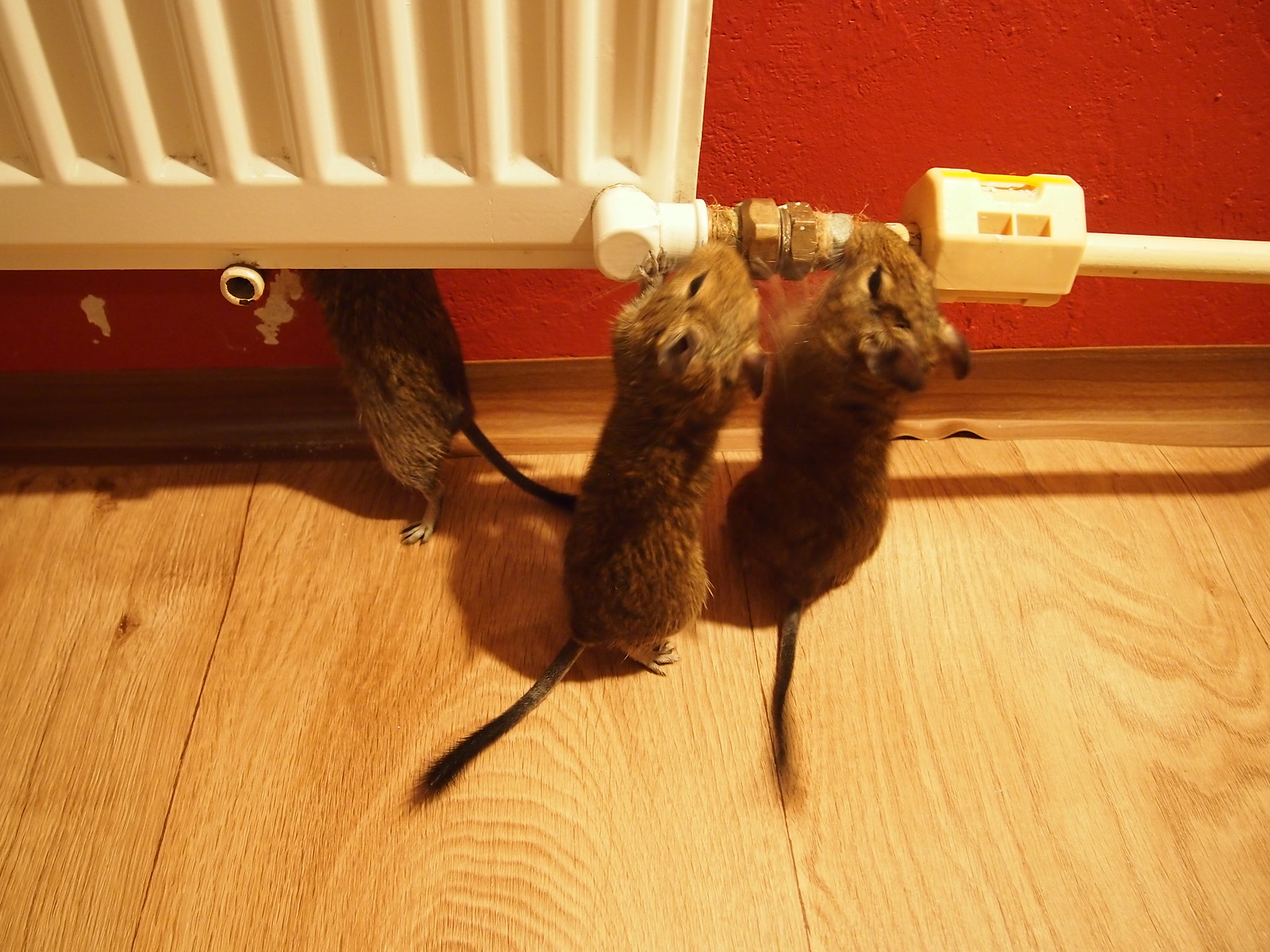The image features a New York apartment with a striking scene of three chestnut brown rodents, possibly mice, engaged in destructive behavior around a wall-mounted cream-colored radiator. The flooring below is a wooden overlay with visible wear, set against a red-painted cement wall showcasing noticeable scratch marks and chipped paint. Two of the rodents are focused on gnawing the connecting pipes and screws of the radiator, while the third rodent, positioned to the left, stands on its hind legs with its head partially obscured behind the heater. Despite the alarming state, the diverse elements of the room – from the radiator's waffle-like design to the rustic wood molding – convey a vivid, albeit unsettling, snapshot of urban living.